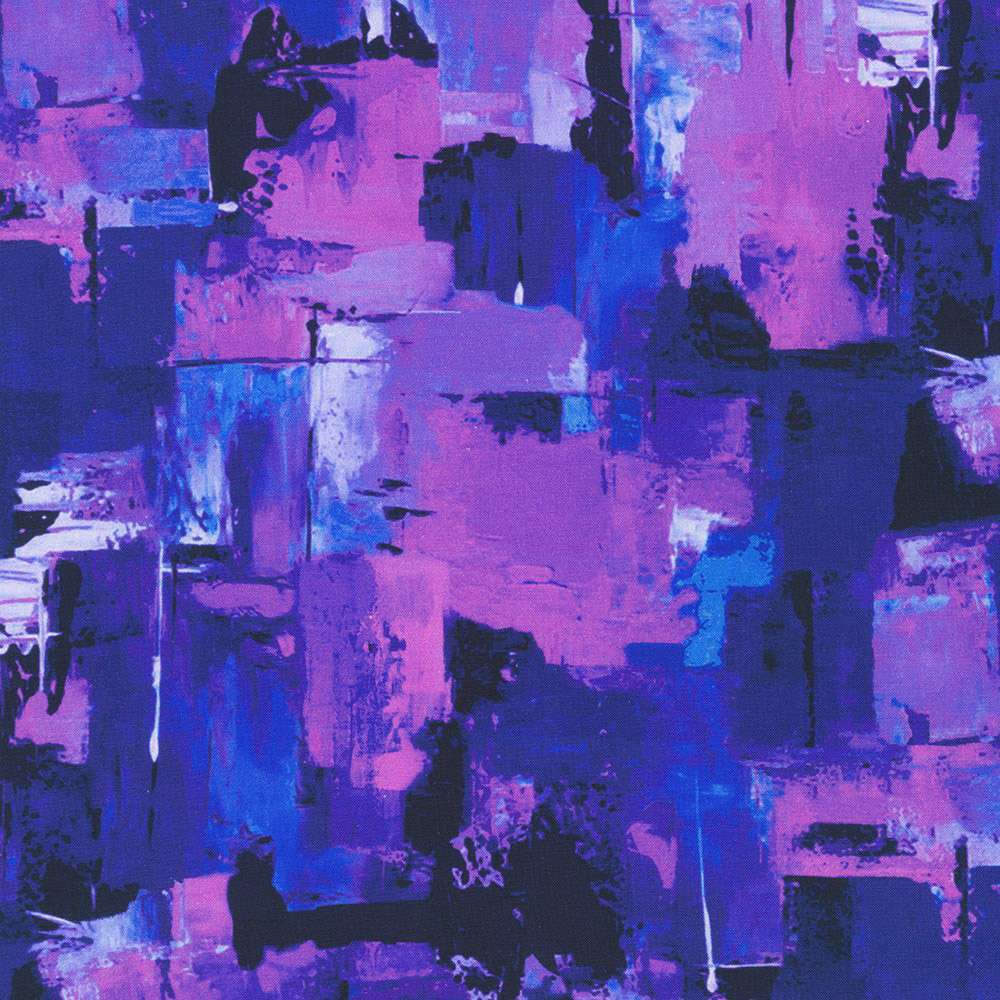This square artwork, captured in a photograph, hovers between digital creation and oil on canvas, though the texture isn't visibly clear. The color palette is dominated by an array of blues and indigos, punctuated by pinks, mauves, black, deep blues, whites, and hints of greyish mauve. This abstract painting employs layers of colors, applied in various directions with both brushes and spatulas. The use of thick brushstrokes contributes to a predominantly linear composition, with the vibrant hues mingling yet maintaining distinct edges. White is strategically used to highlight certain areas. While most shapes within the artwork are rectangular, the overall arrangement is freeform and lacks a specific pattern, encouraging the viewer's brain to discern new patterns with each glance. Some sections appear as splotches with straight edges that blend into adjacent colors, reinforcing the abstract nature of the piece. Though the painting doesn’t depict any recognizable objects, elements within it may suggest abstract forms of furniture or buildings, ultimately leaving interpretation up to the viewer’s imagination.